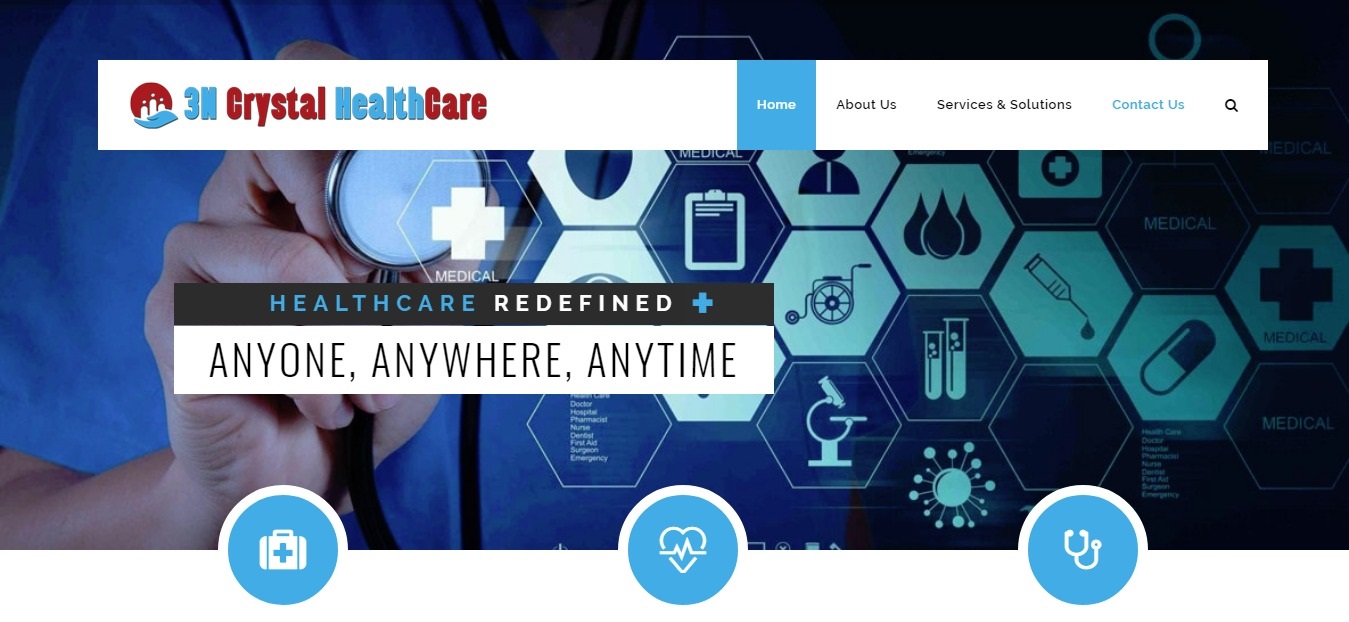The screenshot appears to be the top section of a healthcare provider's website, with a clean, modern design focusing on user-friendliness and visual appeal. The layout is primarily divided into two sections: the top half features a close-up photograph of a healthcare provider, while the bottom half is a blank white background.

The photograph showcases the healthcare provider's right hand holding the stethoscope diaphragm, suggesting a focus on patient care and medical examination. The provider is dressed in short-sleeved blue scrubs, and a small portion of their neck is visible, along with the stethoscope draped around it. The head and the remainder of the provider's body are not visible, keeping the focus on the stethoscope and hand.

Superimposed on this background are several interconnected hexagons, resembling a beehive pattern. These hexagons vary in shades of blue, from dark to light, and each contains a health-related icon. The icons include symbols such as a wheelchair, test tubes, a microscope, a virus, a pill capsule, a first aid cross, and a clipboard, among others. These icons represent various aspects of healthcare and medical services.

At the top of the image, there is a white navigation bar. The left side of this bar has a light blue background with text in red and blue reading, "3H Crystal Health Care" – “Crystal” and “Care” are in red, while the other text is in blue. An icon resembling three white candles on a red circular background accompanies this text. 

In the center of the navigation bar, there's a blue square with the word "Home" written on it. To the right of this home button, there are links labeled "About Us," "Services and Solutions," and "Contact Us," followed by a magnifying glass icon representing a search function.

Additionally, a long rectangular bar is superimposed over the background image with the text "HEALTH CARE REDEFINED." The words "HEALTH CARE" are in blue, and "REDEFINED" is in white. Below this text is a plus sign or black stripe and another white stripe with the text "ANYONE, ANYWHERE, ANYTIME," all in capital letters with commas separating the words.

At the bottom of the website, three bright Carolina blue circles with white icons inside are visible, likely clickable links. These icons represent different functionalities: a first aid kit with a blue cross on it, the outline of a heart with an ECG line, and a stethoscope icon.

This detailed layout suggests a highly organized website design, making it easy to navigate for users seeking healthcare services and information.